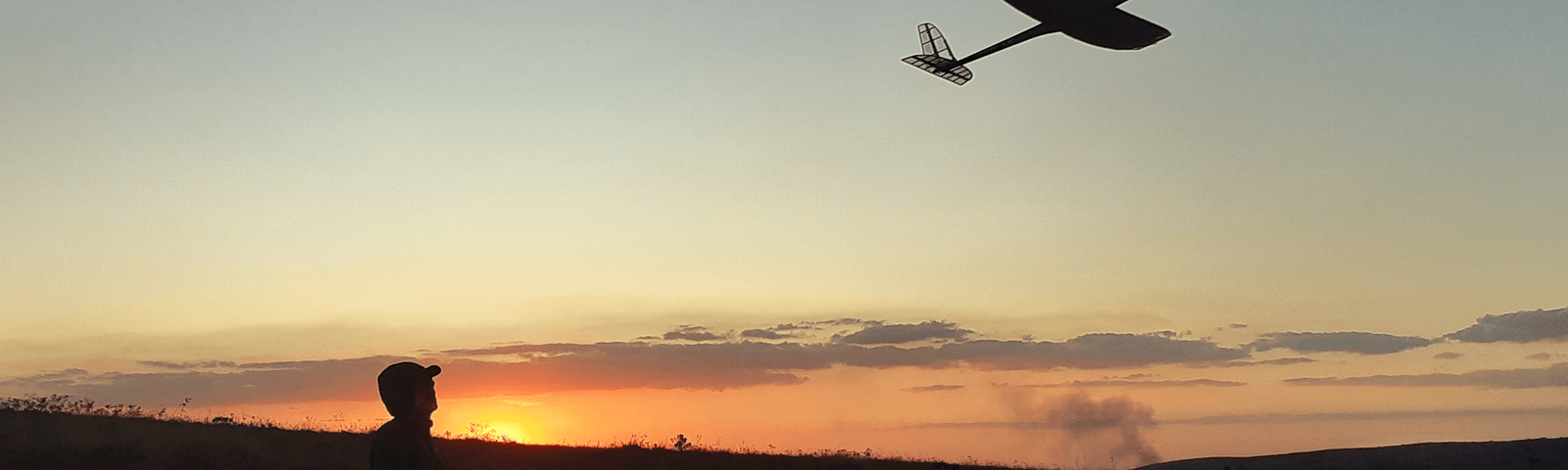A panoramic photograph captures a striking sunset with the sky transitioning from blue to a mix of orange and yellow hues, dotted with wispy clouds. In the silhouette foreground, a man wearing a baseball cap gazes upward towards the right, where a small aircraft resembling a glider or biplane soars through the sky. The terrain below is low-level, without significant mountains, creating a subtle landscape. The sun is descending towards the horizon on the left, casting a warm glow and emphasizing the silhouette of the man's profile and shoulders. The plane, with its distinct tail and side wings, contrasts against the colorful sky, adding depth and intrigue to the tranquil scene.